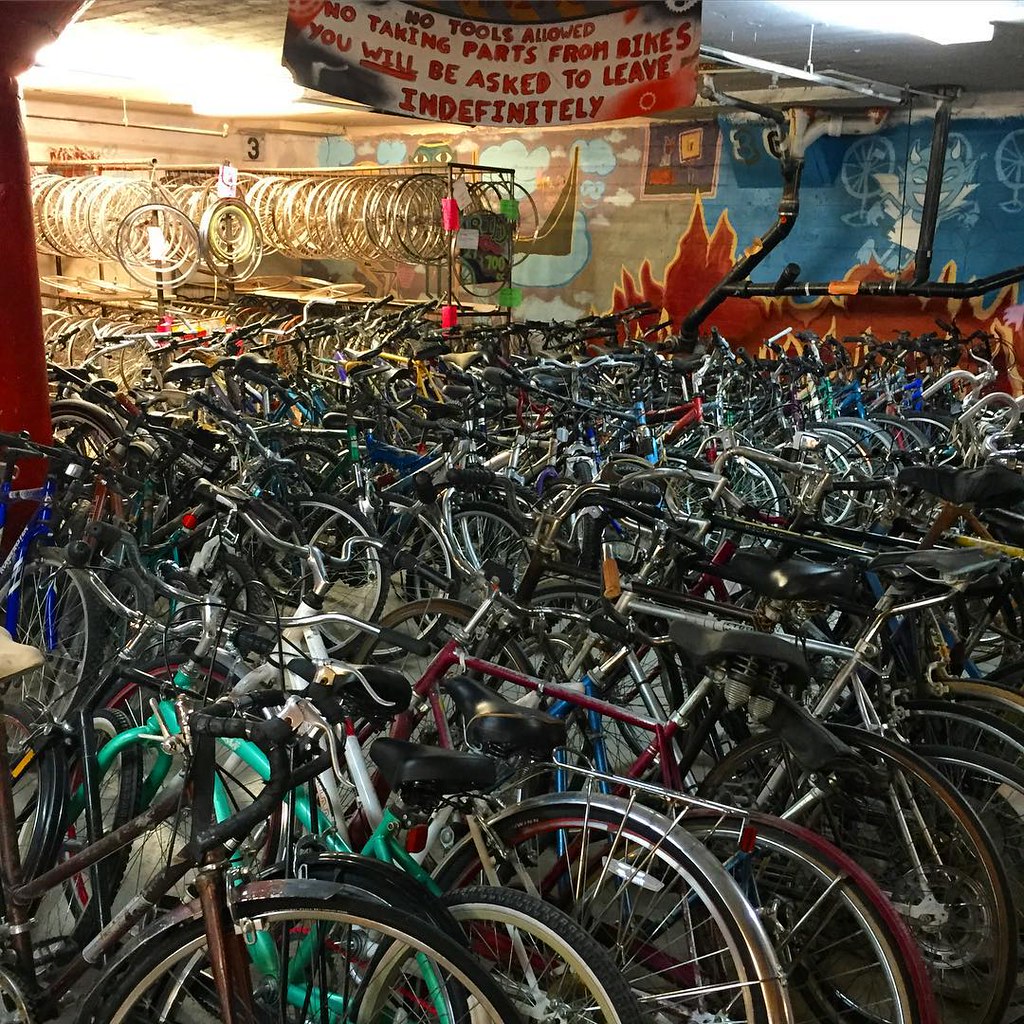The image depicts an incredibly crowded and cramped bike shop filled with what seems to be hundreds of bicycles of all types—mountain bikes, road bikes, small bikes, large bikes, and kid bikes. The foreground is entirely dominated by this chaotic jumble of bikes, stacked in at least two or three rows. In the background, bicycle rims of various sizes hang neatly from racks. The setting appears to be an industrial warehouse or basement, as indicated by visible black pipes, wiring, and mechanical equipment against the concrete walls. These walls are adorned with art, including a vivid mural of a blue devil over fire, among other paintings. A prominent, hand-painted sign with bold red lettering reads: "No tools allowed. No taking parts from bikes. You will be asked to leave indefinitely."